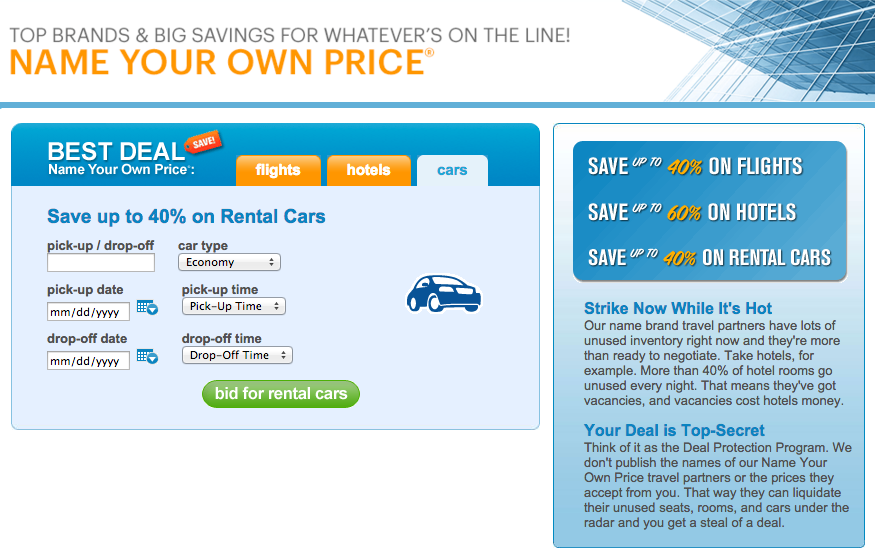This is an infographic sourced from a travel website, showcasing the theme “Top Brands, Big Savings” at the top of the screen in bold letters. Beneath this, the phrase "Name Your Own Price" is prominently displayed in bright orange. Directly underneath, there's a blue tab with an elongated blue line for visual separation.

At the top of the infographic, there is a side profile image of a skyscraper, adding visual interest and context. Below this image, two distinct information boxes are presented.

The first box highlights rental car deals with the headline, "Best Deals Name Your Own Price for Car Rentals." It mentions potential savings of up to 40% on rental cars. This section includes options for selecting pick-up and drop-off locations, car type (specifically economy), along with notifications for pick-up time and date.

On the right-hand side of the screen, the second box details additional savings: up to 40% on flights, up to 60% on hotels, and similarly up to 40% on rental cars. This section encourages urgency with the phrase, "Strike Now While It's Hot." It explains that name-brand partners have a surplus of unused inventory and are keen to negotiate. For example, more than 40% of hotel rooms remain vacant each night, indicating substantial opportunities for savings.